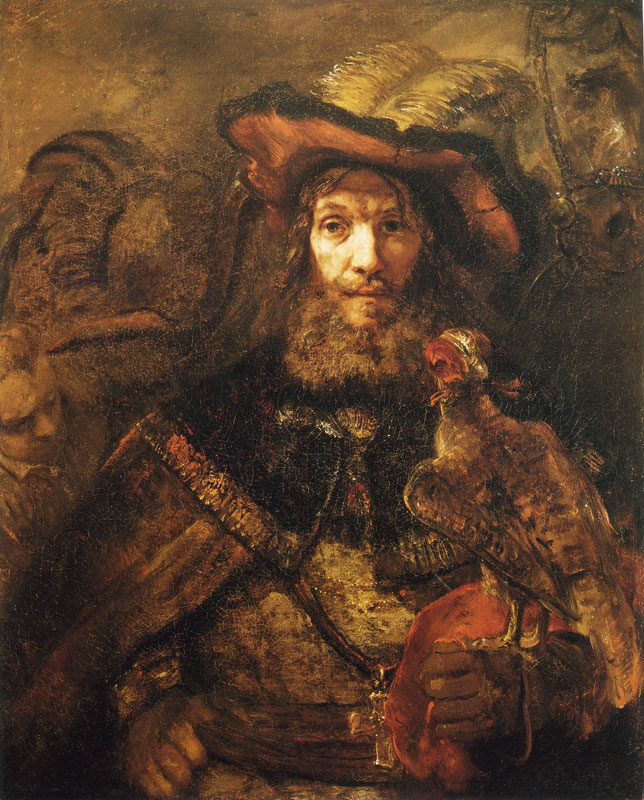The painting depicts a bearded white man with a prominent bushy reddish-brown beard and a mustache, dressed in elaborate Renaissance attire. His outfit includes a long, thick, dark brown coat adorned with intricate golden patterns and a flat, floppy hat embellished with two large white feathers. He also wears a necklace with a cross that hangs down to his waist. The man, possibly a falconer or warrior, stands centered in the frame, gazing slightly to the left of the viewer. In his gloved left hand, perched on the right side of the image, is a bird of prey, likely a falcon, with its back to us. The background is dominantly brown, illustrating a textured wall with subtle human faces and figures. An orange handkerchief is draped over his hand, complementing the brown and orange tones prevalent throughout the painting. Additionally, some faint human figures or shadows appear in the background, enhancing the historical ambiance.